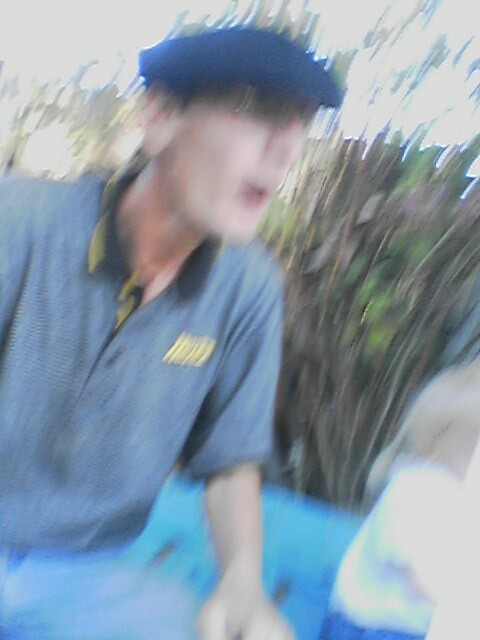In this slightly out-of-focus photograph, a man is seated outdoors amidst an indiscernible backdrop of greens and browns, suggesting a natural setting, possibly during a picnic. The sky above appears pale and overcast. The man, a Caucasian with short brown hair mostly concealed under a dark blue beret, sports glasses. He is dressed in a blue-gray polo shirt with a navy blue and yellow collar, adorned with yellow text on the left breast. His attire includes vintage-style blue jeans reminiscent of the 1980s. The man’s left arm is visible, crossing over his legs, hinting at a relaxed posture. In the foreground, partially hidden, a toddler with longish blonde hair is visible. The child wears a pale shirt and vibrant royal blue jeans, adding a splash of color to the scene.